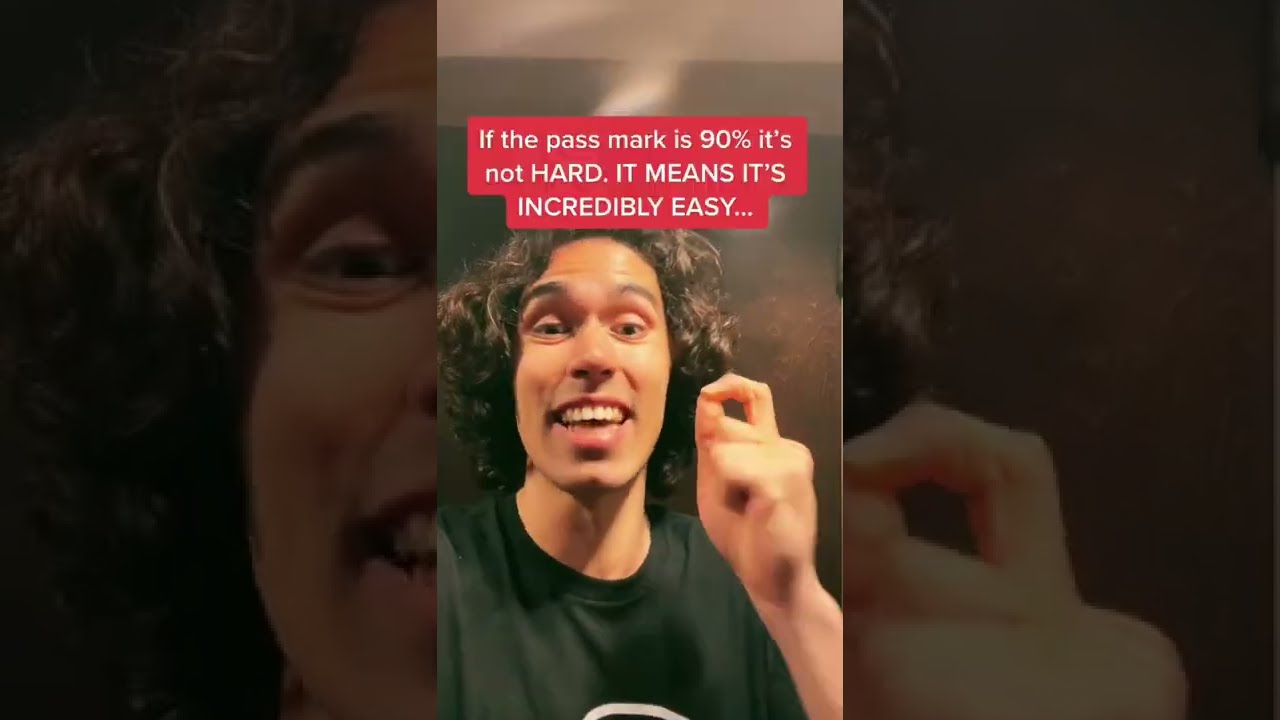The image is a pre-paneled photograph, divided into three sections. The central panel prominently features a man with short, bushy, dark brown wavy hair that reaches the back of his neck. He is wearing a black t-shirt, which appears to have a white logo or drawing. His slightly dark Caucasian skin contrasts with his straight, white teeth as he smiles, mid-speech, or as if about to say something. His left hand is raised in front of him, his thumb and pointer finger forming an 'O', while the rest of his fingers are in a relaxed fist, emphasizing his gesture.

The left and right panels are darker, close-up versions of the central image from different angles. The left panel highlights the left side of his face and hair, whereas the right panel shows the end portion of his hair and his clasped fingers. 

Above his head in the central panel, there is text bordered in red with bold, white letters that states: "if the pass mark is 90% it's not hard it means it's incredibly easy." The words "hard" and "it means it's incredibly easy" are all in capital letters, with "incredibly easy" trailing off with an ellipsis (...) for added emphasis.